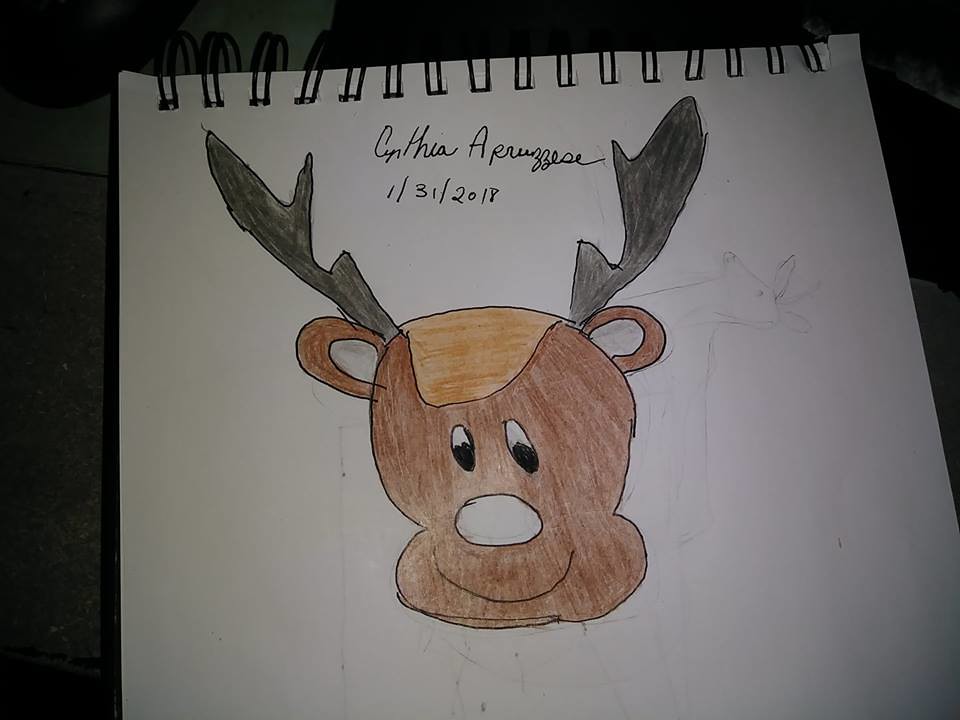This close-up photograph captures a colorful, cartoonish drawing of a reindeer, likely created by a child named Cynthia. The drawing is on a white sketch pad with coiled binding at the top, filled mostly with blank sheets. The reindeer is illustrated in shades of brown with black antlers and a prominent, uncolored nose. Its eyes have black pupils, suggesting a lively expression, and there are ears underneath the antlers with gray insides. The reindeer sports a simple line smile. The child has signed her name, albeit a bit sloppily, above the drawing as "Cynthia" with a surname that's difficult to decipher. The date, handwritten as "1-31-2018," accompanies the signature. The drawing media includes colored pencils and possibly crayons. In the background, faint traces of an erased pencil sketch add a layer of depth to the notepad.